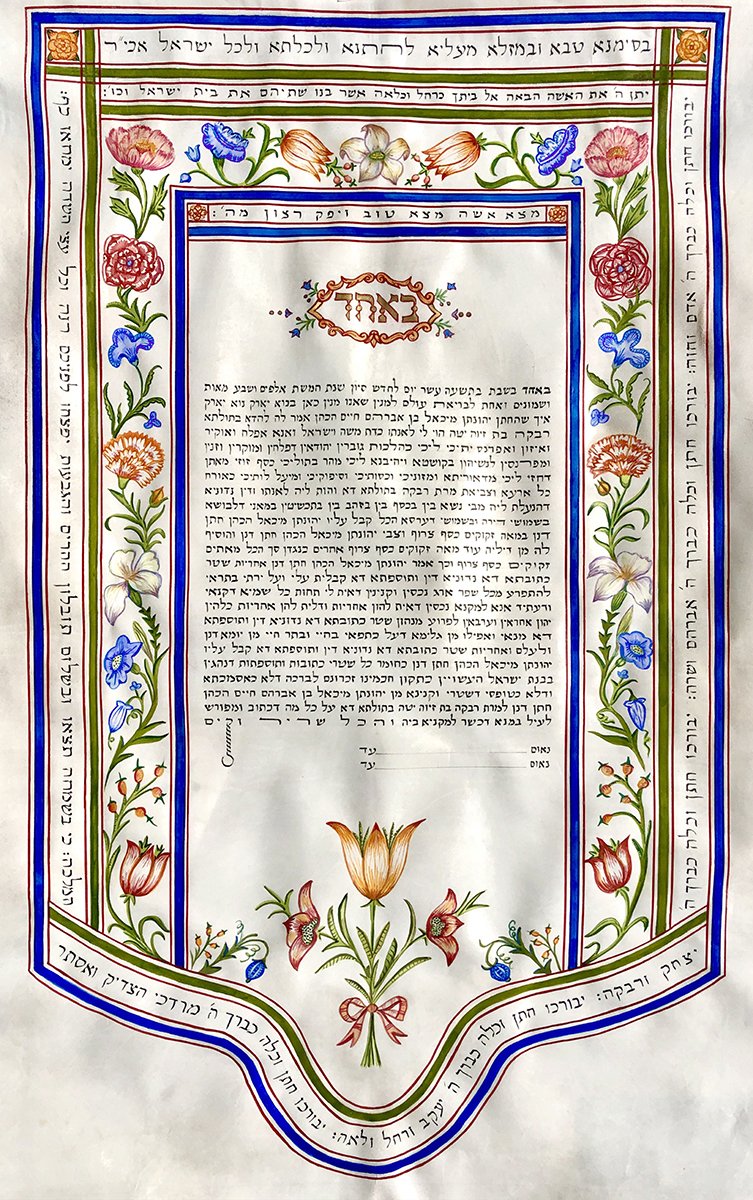This image depicts a fabric banner, likely silk, adorned with intricate and symmetric details. The design features multiple borders, starting with a red outline, followed by a quarter-inch thick blue border, another thin red line, and a green border, each outlined by thin red lines. The main section of the banner is filled with ornate flowers, including orange tulips, red roses, and white marigolds. These flowers are meticulously arranged with bilateral symmetry around a central block of text, believed to be in Hebrew or possibly Yiddish, which remains unreadable to the viewer. The text is also present along the border, extending around the banner’s entire perimeter. The overall shape of the banner is portrait-oriented, with the bottom featuring a distinctive curved dip that arcs and then dips further in the center, adding a unique touch to its design.